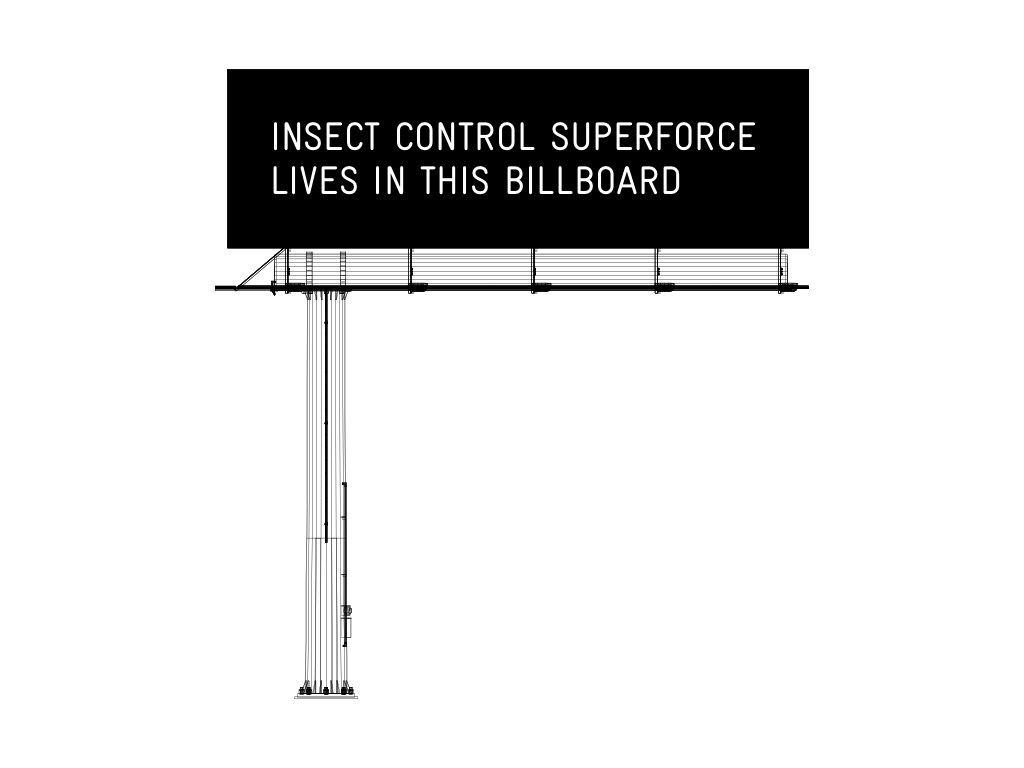A metal structure stands rigidly upright, resembling a billboard with an intriguing message. The top section displays the text "INSECT CONTROLS THE SUPER FORCE, LIVES IN THIS BILLBOARD" in bold, capital letters, centered for emphasis. Above the text, there are white bars and railings, suggesting a platform that could potentially support a person. To the left side of the structure, a vertical metal pole with noticeable ridges extends upward, accompanied by a black pipe attached to its side. The front of the structure features additional black pipes. At the base, the pole is securely bolted to a square foundation that is firmly fixed to the ground.